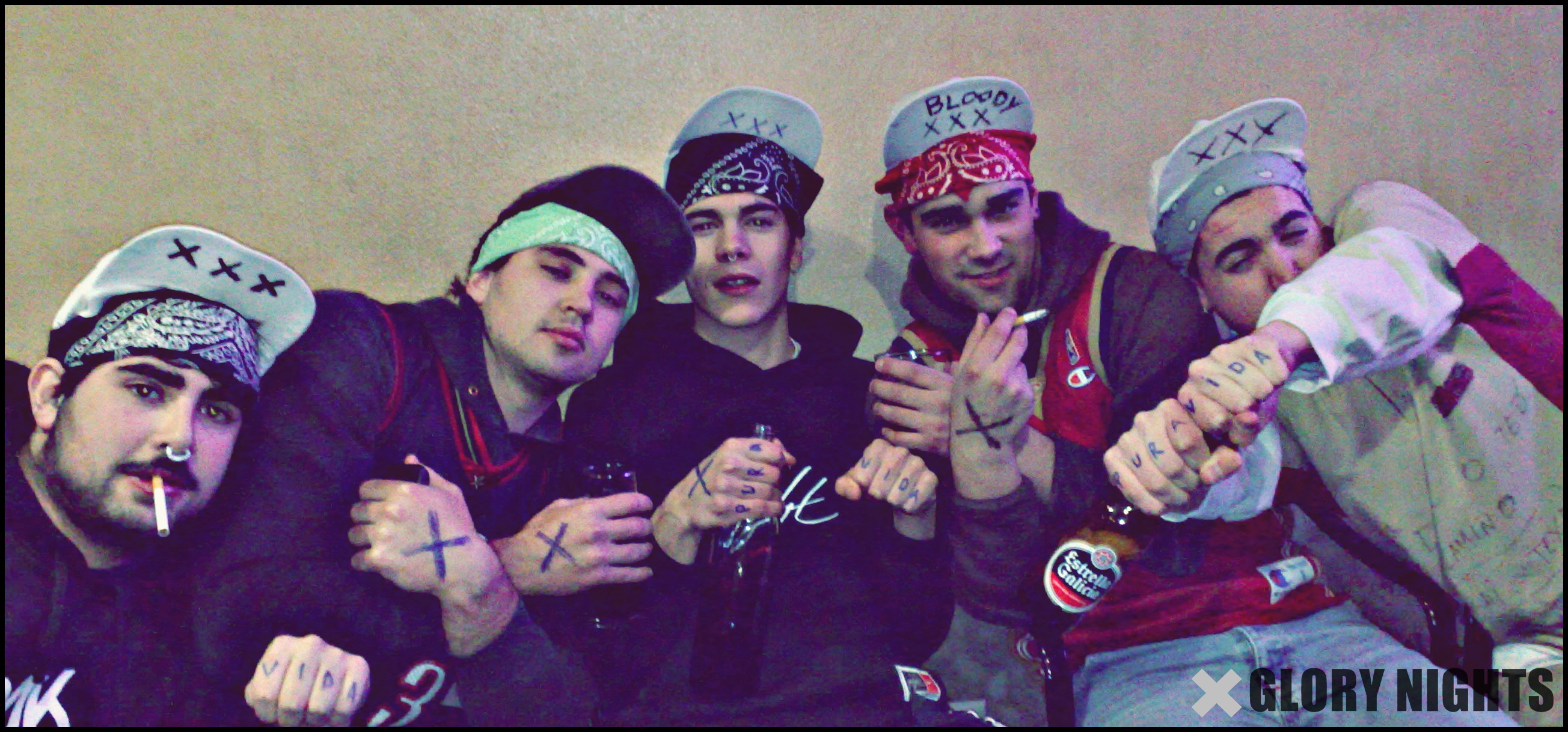The photograph features five young men dressed in hip-hop style attire, standing close together against a solid gray background. In the bottom right corner of the image, the words "Glory Nights" are displayed in black text, along with a gray X to its left. The men are posed from left to right as follows:

1. The first individual, partially visible from the shoulders up due to the angle, wears a white baseball cap with three black X's marked under the bill, a black and white bandana underneath, and a black hoodie. He sports a mustache, beard, a silver nose ring shaped like a rose, and has an unlit cigarette in his mouth.
  
2. Standing next to him is a person in a black and red sleeveless basketball jersey over a black hoodie, wearing a green and white bandana with a black baseball cap. His hands, crossed in front of him, display drawn X's.

3. The central figure, wearing a white baseball cap with "bloody" and three X's written under the brim, a blue bandana, and a navy hoodie, has "Pura Vida" tattooed across his knuckles. His concealed shirt features white writing, and he is holding a bottle or making a fist.

4. To his right stands a man also with a white cap marked with three X's and a red bandana. He wears a Champion brand jersey, a navy hoodie, and jeans, holding a lit cigarette in one hand with an X on his hand.

5. The rightmost individual dons a white hat with three X's, a light blue bandana, and holds his arms up showing "Pura Vida" tattooed on his knuckles. His white and red color-blocked shirt has handwritten words including "Ted," "Camino," and "Texas."

Together, they create a unified yet detailed representation of their shared style and camaraderie.